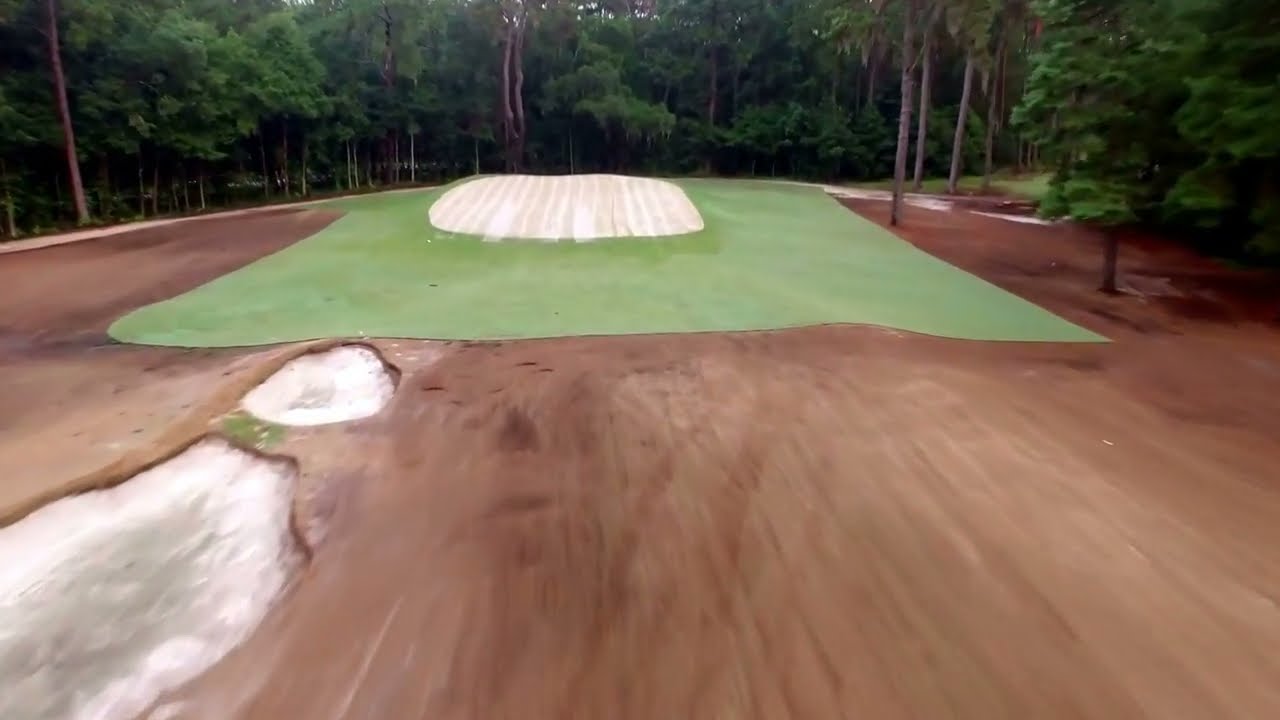The photograph depicts a golf course under construction, featuring a large expanse of brown dirt with a distinct green square section positioned centrally. This green area contrasts sharply against the surrounding dark brown soil. In the middle of the green section, there is a prominent white mound, marked with brown lines. On the bottom left of the dirt section, there are two dugouts: one lighter gray and white situated slightly to the center, and a smaller, whiter gray one positioned just in front. The background is enveloped by a dense forest of tall trees with dark green leaves and visible brown trunks, creating an impenetrable green wall around the dirt course. The viewpoint provides a sense of movement, as if captured from a rider on a bike or motorcycle, heading towards the green area amidst the forested surroundings.